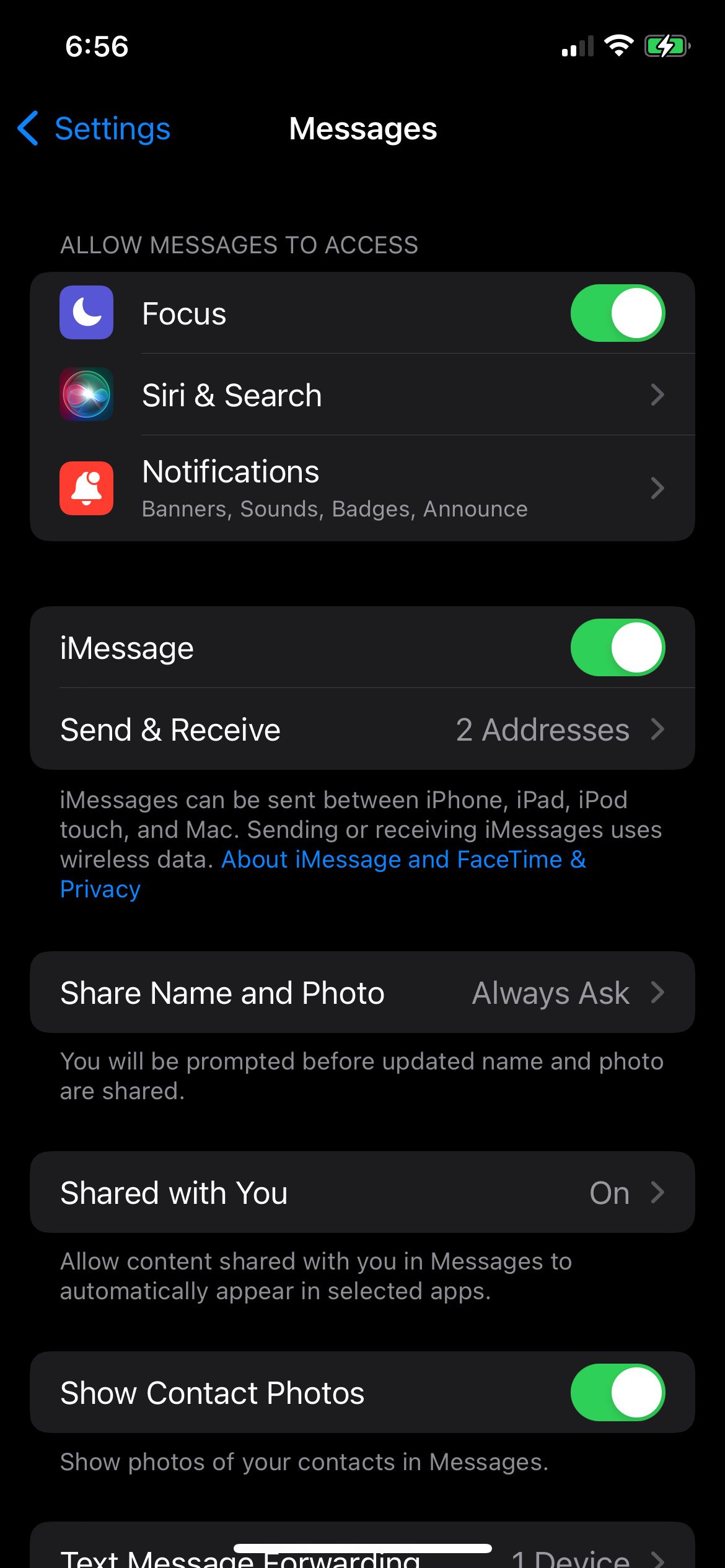A detailed caption for the image could be:

"This screenshot, captured on a mobile device such as an iPhone or iPad, shows the screen at the timestamp of 6:56 AM. The device has three bars of service, full Wi-Fi connectivity, and a fully charged battery. The image specifically displays the 'Messages' settings section. At the top left, there's a back arrow allowing the user to exit the settings. Various 'Allow Messages to Access' options are visible, including 'Focus', which is toggled on, 'Siri & Search', and 'Notifications'. Under the 'Notifications' setting, it specifies 'Banners, Sounds, Badges, Announce'. The iMessage feature is activated with 'Send & Receive' set to two email addresses, indicating iMessages can be sent and received on two accounts. It is mentioned that iMessages can be sent between iPhone, iPad, iPod touch, and Mac devices, and that using iMessage will consume wireless data. There's information on 'About iMessage and FaceTime Privacy'. The 'Share Name and Photo' option is configured to 'Always Ask', meaning the user will be prompted before their name and photo are shared. The 'Shared with You' feature is enabled, allowing content shared within messages to automatically appear in selected apps, and 'Show Contact Photos' is also toggled on."